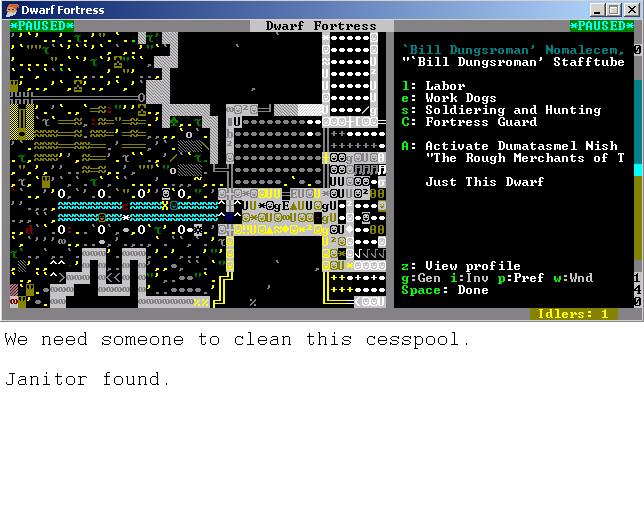This image showcases a screenshot of the classic 2D computer game "Dwarf Fortress," displayed within an old-school Windows interface, identifiable by the characteristic blue title bar and Windows control icons (minimize, maximize, close) at the top right. In the upper left, the blue bar prominently reads "Dwarf Fortress," alongside an icon depicting a dwarf. The upper corners of the game window feature the word "Paused" in green text, emphasizing that the game is not in progress.

Dominating the left two-thirds of the screen is a maze-like game environment, rendered in a highly pixelated, blocky style reminiscent of early computer graphics, with a mixture of ASCII characters, dots, and blocks suggesting various elements of the game world. 

The right third of the screen is dedicated to a message log and command shortcuts, all set against a black background. The log includes various instructions and game messages such as "Bill Dung's Roman Staff Tube," alongside keyboard shortcuts labeled for different game functions: L for Labor, E for Work Dogs, S for Soldiering and Hunting, C for Fortress Guard, A for Activate, and Z to View Profile. Additional commands like GGen, Iinv, Ppref, and W Window hint at functionalities within the game, with "Space" being used to finalize selections (as indicated by "done").

At the very bottom of the screen, crucial game text reads, "we need someone to clean this cesspool. Janitor found," indicating a current task or event in the game. The backdrop and overall color scheme of the game use predominantly black, white, blue, green, and yellow hues, embedding it firmly in the aesthetics of early computer games.